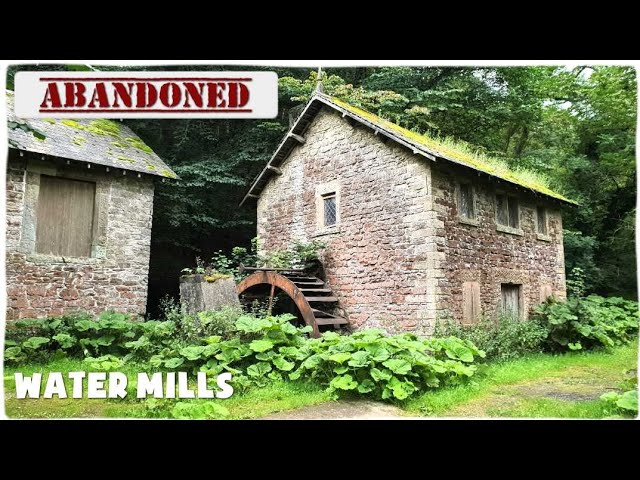The image depicts an abandoned, dilapidated watermill, prominently featuring a notification in the top left corner with a white square and red lettering stating "ABANDONED," and the label "watermills" at the bottom. The primary structure centers on an old stone building to the right, its windows boarded up, and a decaying wooden roof laden with moss and grass indicating long-term disuse. Attached to its left is a deteriorating water wheel, enshrouded by dense vegetation. Another partially visible stone building to the left similarly exhibits signs of abandonment, with its boarded-up window and roof covered in green moss. Both structures are encircled by lush foliage and trees, suggesting an overgrown woodland setting that further accentuates the scene's historic and forsaken character. Overall, the weathered stone walls and extensive plant growth convey a picturesque yet melancholic image of enduring but forgotten architecture.